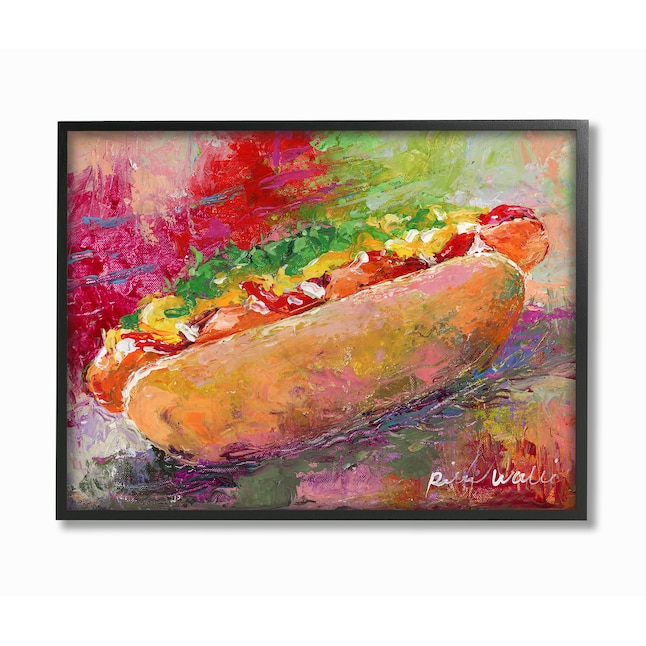The image is a striking and vibrant piece of digital art, designed to emulate a highly textured, abstract oil painting of a hot dog. Encased in a black frame with an artificial drop shadow, the hot dog sits prominently in the center of a colorful canvas. The background is a riotous blend of rainbow watercolors, featuring splatters and gradients of green, red, yellow, blue, pink, purple, brown, orange, and gray, creating a chaotic yet mesmerizing backdrop. 

The hot dog itself is depicted in a large bun and presented with a variety of toppings. The hot dog is a vivid orange color, adorned with red ketchup, yellow mustard, and green relish, which are applied in loose, colorful swirls. There are also small bits of white onion sprinkled on top, although the quantity is minimal. The bun is similarly colorful, with splashes of pink, yellow, gray, and orange as if the colors from the background have bled into it. 

In the bottom right corner of the painting, there is an indiscernible artist's signature, possibly beginning with an "R" or "P" for the first name and a "W" for the last name. Overall, this piece is a vibrant, loose, and textured abstraction of an ordinary hot dog, making for an interesting and unconventional subject matter.